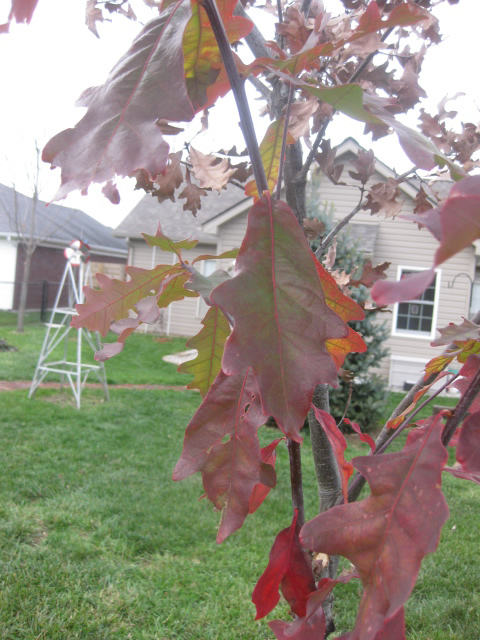In this detailed and slightly hazy outdoor photograph, the central focus is a close-up shot of an autumnal tree branch with drooping, large purplish-orange leaves, transitioning from their original green hue. The branch is set in the foreground of what appears to be someone's yard. Behind the vibrant leaves, lush green grass is visible, along with a small white windmill or wind sock adding a quaint touch to the scenery. To the right, a brown garage with a white door and a gray roof can be seen, adjacent to a house with tan siding and a rectangular window framed in white. Further adding to the charm, a shepherd's hook stands on the far right, and a small pathway leads from the house, which has a gray peaked roof, extending out of the frame on the left. The scene also includes a tall, skinny tree and a smaller pine tree in the background.